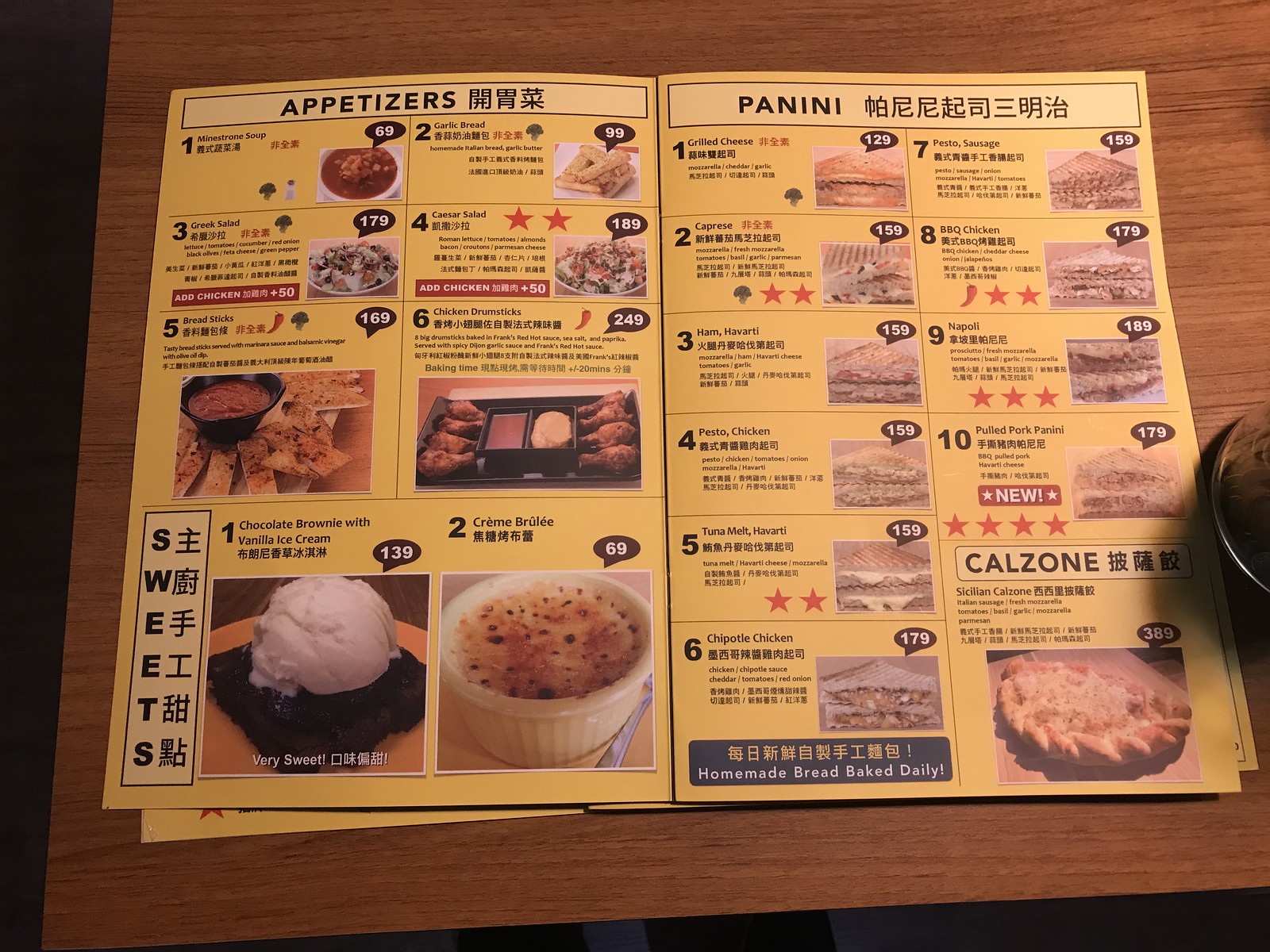The image features an open menu displayed on a wooden-colored desk. The menu appears to be written in Korean and is opened fully upwards, offering a clear view of its contents. 

On the left pane of the menu, the heading "Appetizers" is written in black leather, accompanied by Korean characters. Beneath this heading, the appetizer items are listed sequentially from one to six, each presented in individual boxes with short descriptions also in Korean. 

Further down, there is a section labeled "Sweet," containing two items: a chocolate brownie with vanilla cream and a crème brûlée, each identified by numbers one and two.

On the right side of the menu, the heading "Paninis" is displayed, followed by corresponding Korean text. This section lists ten different types of sandwiches, numbered sequentially from one to ten. 

At the bottom of the right pane, there is an additional section dedicated to calzones.